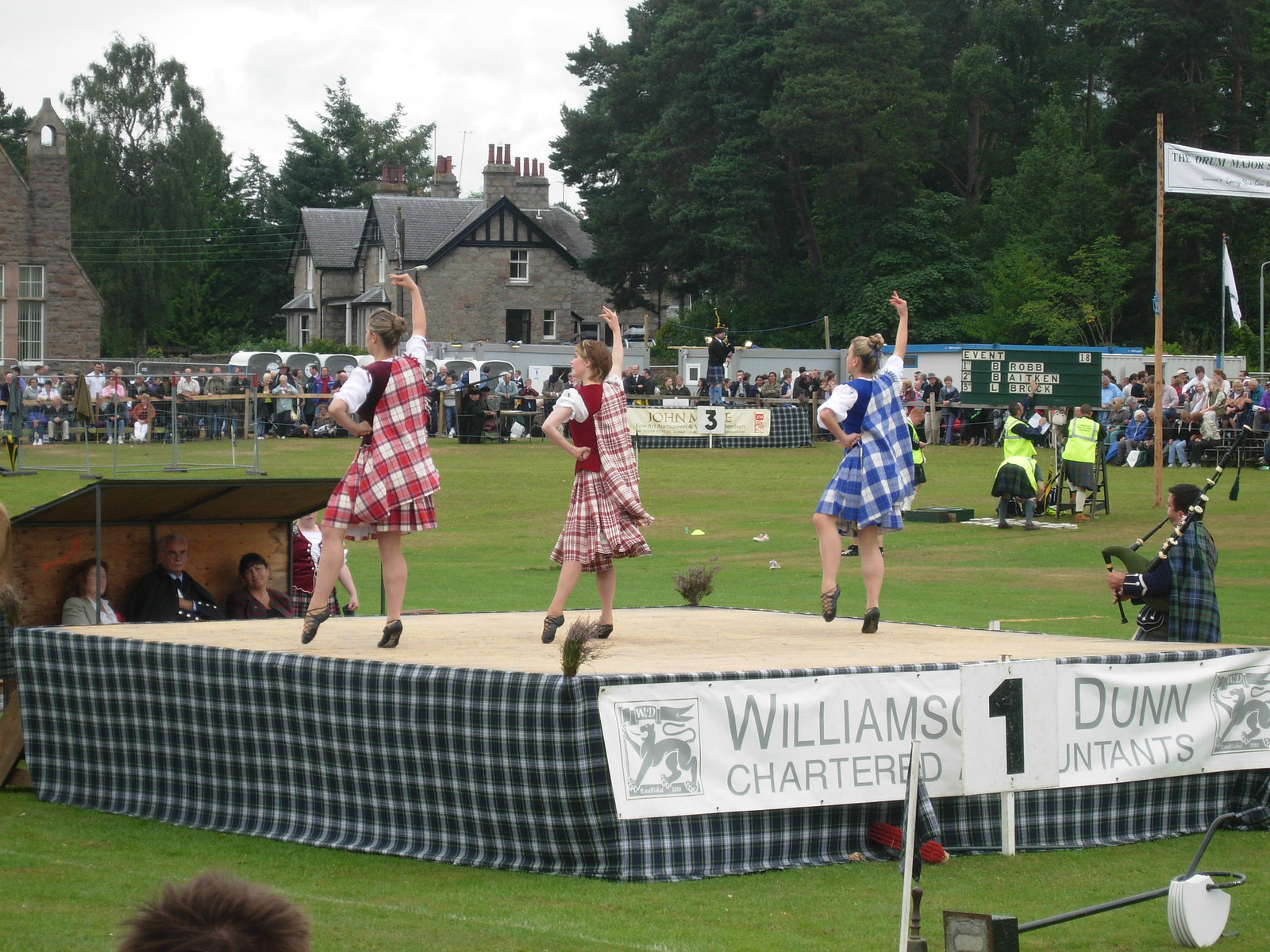In the image, three girls stand on a well-decorated stage, presumably participating in a Scottish or Irish dance competition. The stage features a green and white plaid cloth draped around its base, concealing the structure underneath. The girls are attired in traditional outfits: two wear red and white plaid skirts, while the third sports a blue and white plaid skirt. Each girl complements her skirt with a matching vest worn over a white shirt. A prominently displayed sign on the stage reads "Williams Dunn Chartered," though the last word remains partially obscured by the large number one positioned next to it.

The event takes place outdoors in a spacious, grassy field, with a sizable crowd of spectators gathered to watch. In front of the stage, three individuals are seated in a small, roofed structure resembling a lean-to with an open front and sides. They likely serve as judges, attentively observing the dancers who have their backs turned to the camera. The vibrant atmosphere is filled with the presence of family, friends, and onlookers, all seemingly enjoying the event amidst a picturesque backdrop.